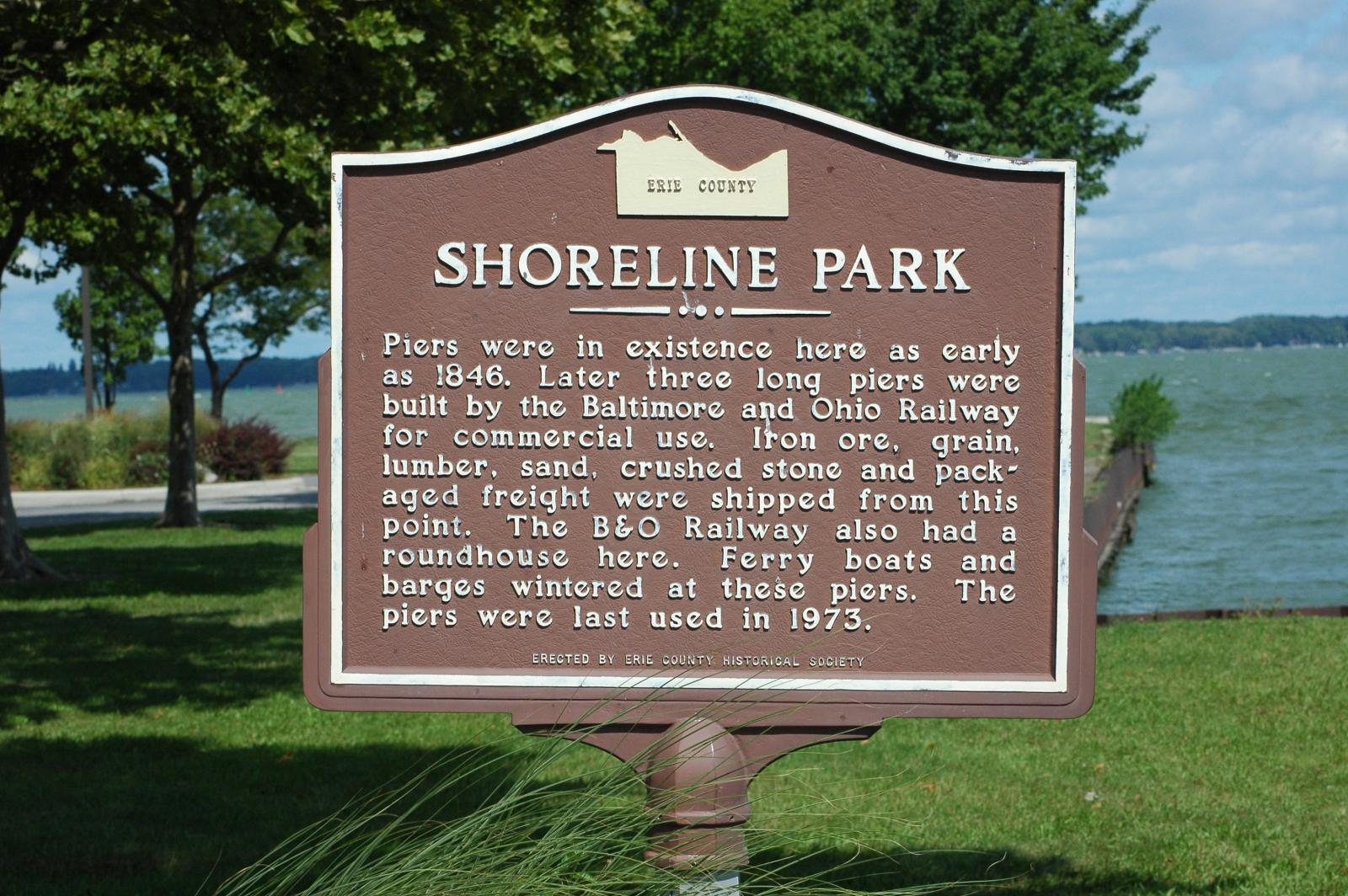In this outdoor scene at Shoreline Park, the large brown sign with white lettering stands prominently against a backdrop of a serene lake with bluish-green water, under a sky dotted with puffy white clouds. The well-manicured, lush green grass stretches out in the foreground, complemented by the verdant foliage of nearby trees. The sign, perched atop a pole, reads:

"Shoreline Park  
Piers were in existence here as early as 1846. Later, three long piers were built by the Baltimore and Ohio Railway for commercial use. Iron, ore, grain, lumber, sand, crushed stone, and packaged freight were shipped from this point. The B&O Railway also had a roadhouse here. Ferry boats and barges wintered at these piers. The piers were last used in 1973."

At the bottom, it is noted that the sign was "Erected by Erie County Historical Society," marking the site’s historical significance.